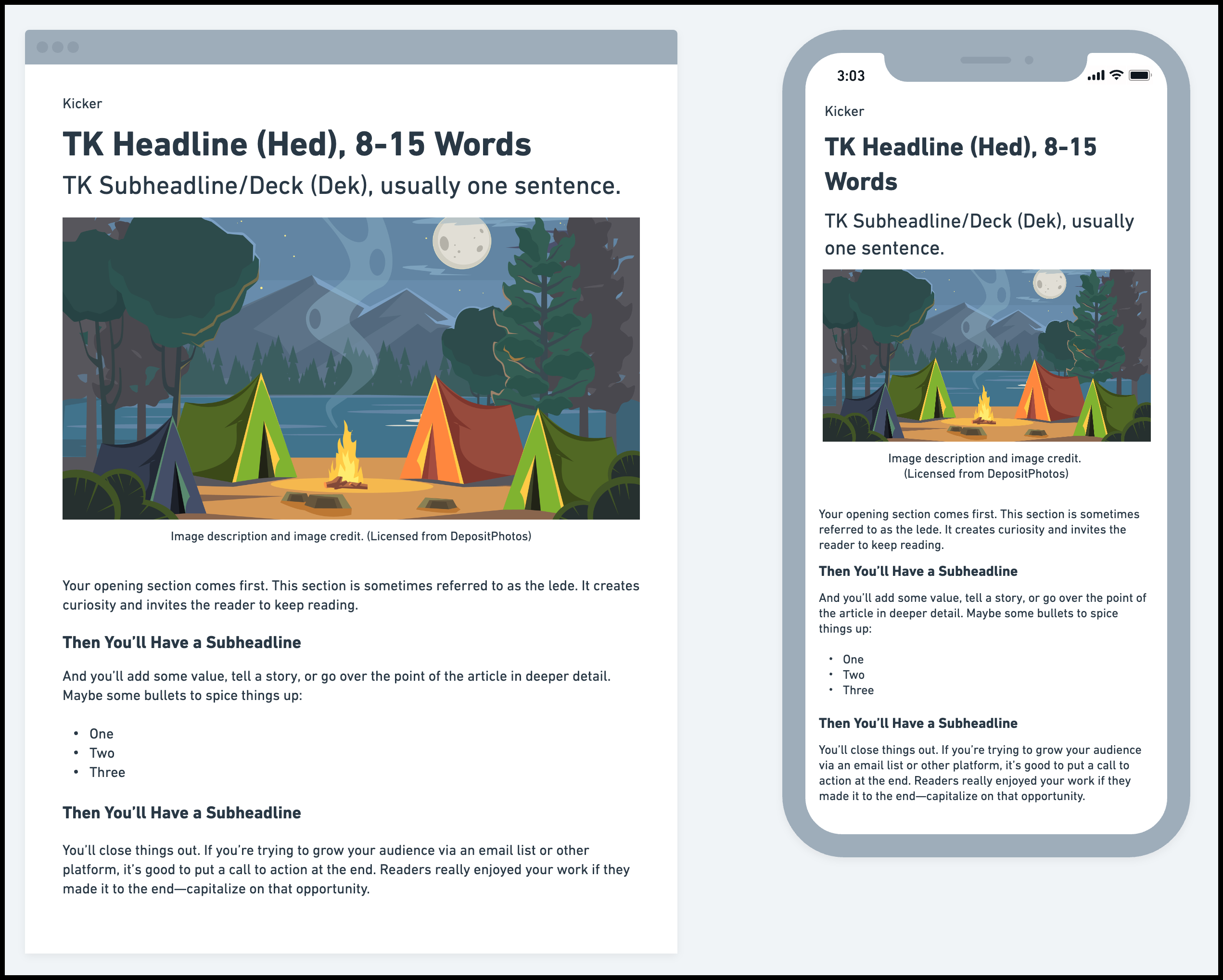This image showcases a side-by-side comparison of a sample website layout as it appears on both a computer browser and a mobile phone. The template, possibly named "Kickr," features placeholder text to help users visualize their content. At the top of the template, there's a placeholder for the main headline, "TK headline, 8-15 words," followed by a subheadline, "TK subheadline / deck, usually one sentence."

Below the text placeholders is a striking illustrated image depicting four tents—blue, green, orange, and another green—arranged around a campfire by a lakeside, surrounded by trees at night. The image description mentions that the illustration is licensed from Deposit Photos.

Further down, the layout includes sample text elements such as a subheadline, bullet points, paragraphs, and additional subheadlines, providing users with a comprehensive preview of how their website or article would appear using this template.